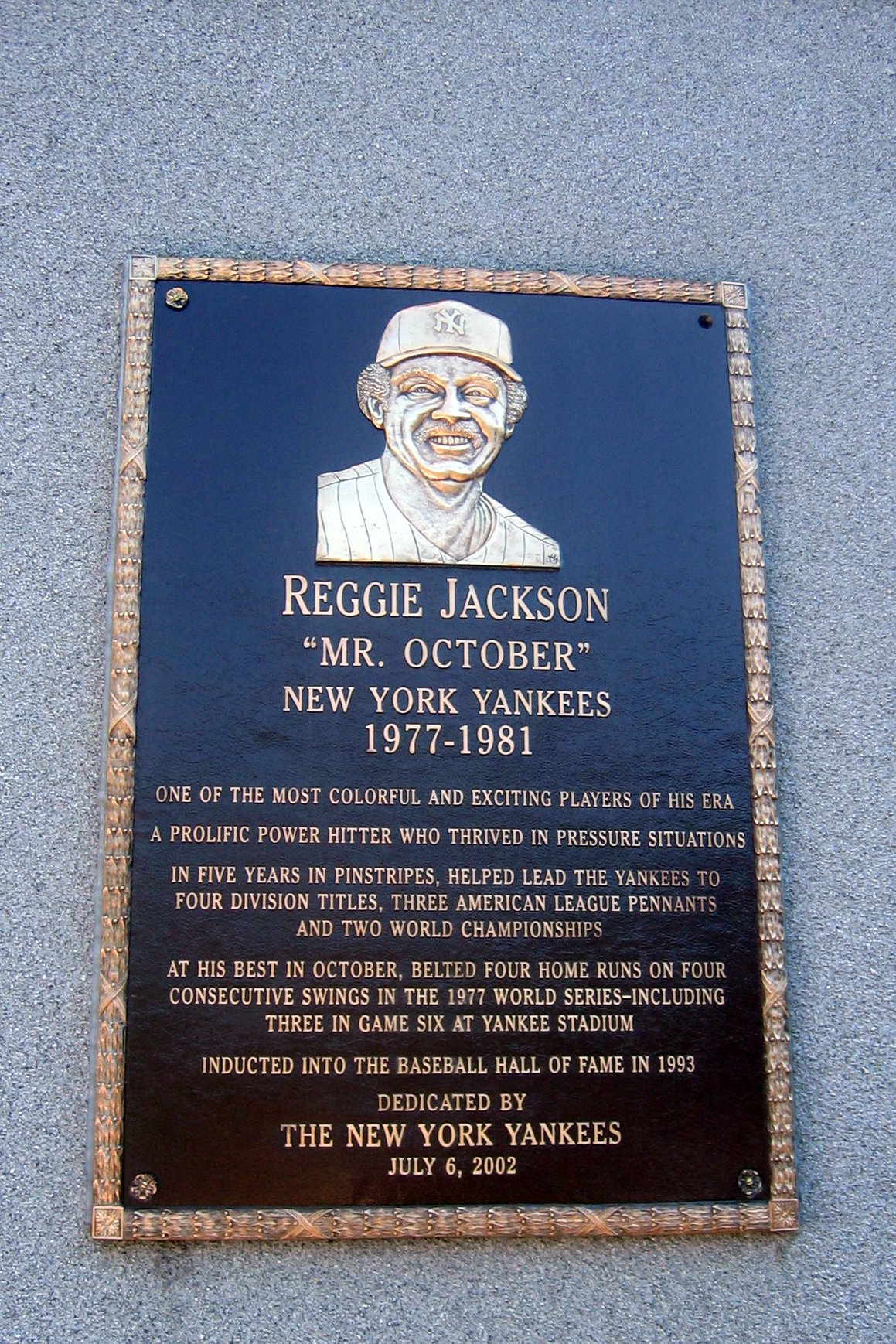The image showcases a detailed plaque dedicated to Reggie Jackson, nicknamed "Mr. October," prominently framed in gold or bronze with a black background. At the top of the plaque, there is a metallic depiction of Reggie Jackson's face. Below the image, the plaque reads his name "Reggie Jackson," followed by his nickname "Mr. October," and his tenure with the New York Yankees from 1977 to 1981. The text beneath commemorates Jackson's remarkable achievements, highlighting him as one of the most colorful and exciting players of his era, noted for his prolific power hitting and ability to excel in high-pressure situations. During his five years with the Yankees, Jackson helped the team secure four division titles, three American League pennants, and two World Series championships. Notably, he hit four home runs on four consecutive swings in the 1977 World Series, with three of those home runs occurring in game six at Yankee Stadium. Reggie Jackson was inducted into the Baseball Hall of Fame in 1993, and this plaque, dedicated by the New York Yankees, was installed on July 6, 2002.